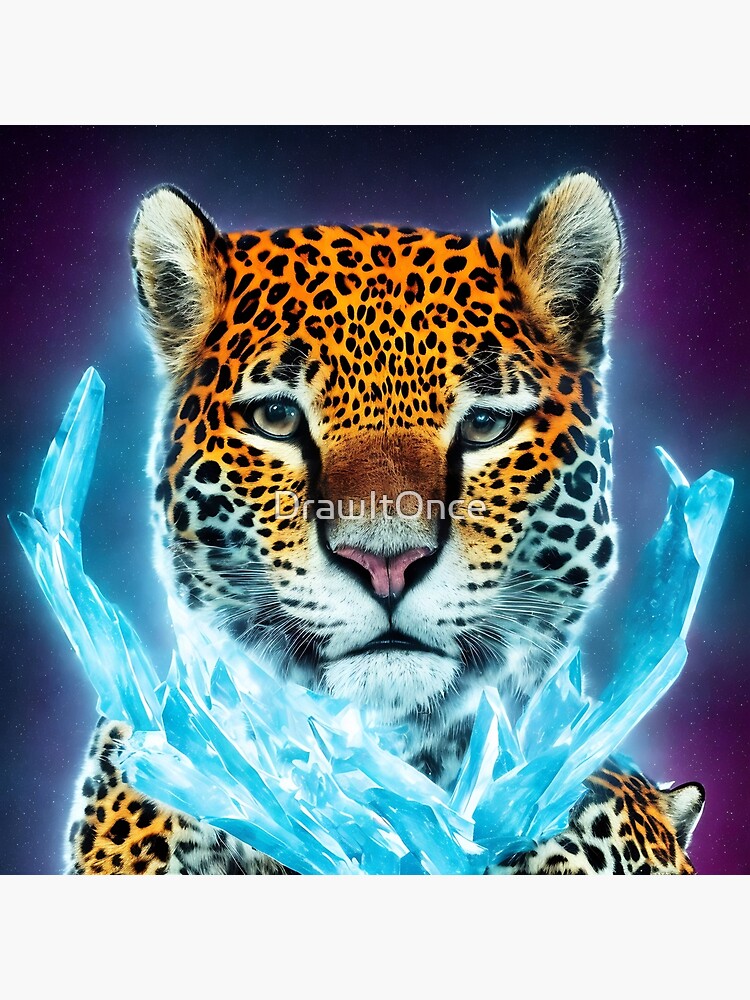This detailed color illustration presents a captivating fantasy portrait of a Bengal tiger. The square-format image centers on the tiger's face, visible from the top of its ears to mid-neck, positioned directly facing the viewer. The tiger's coat is a striking blend of orangish-beige fur marked with various sized black spots, transitioning to white around its snout, cheeks, and the inside of its small, rounded ears. It boasts mesmerizing light green eyes, a pink nose, and prominent white whiskers. The background of the illustration blends from a dark bluish-purple to a softer violet, creating a mystical atmosphere. Encircling the tiger's face are two translucent, blue crystal-like formations that resemble ice sculptures, adding a surreal and enchanting effect. The entire scene is bathed in a soft, glowing light that outlines the tiger in an ethereal white glow. Across the tiger's nose, a subtle photo credit, "draw it once," is elegantly inscribed in white text.